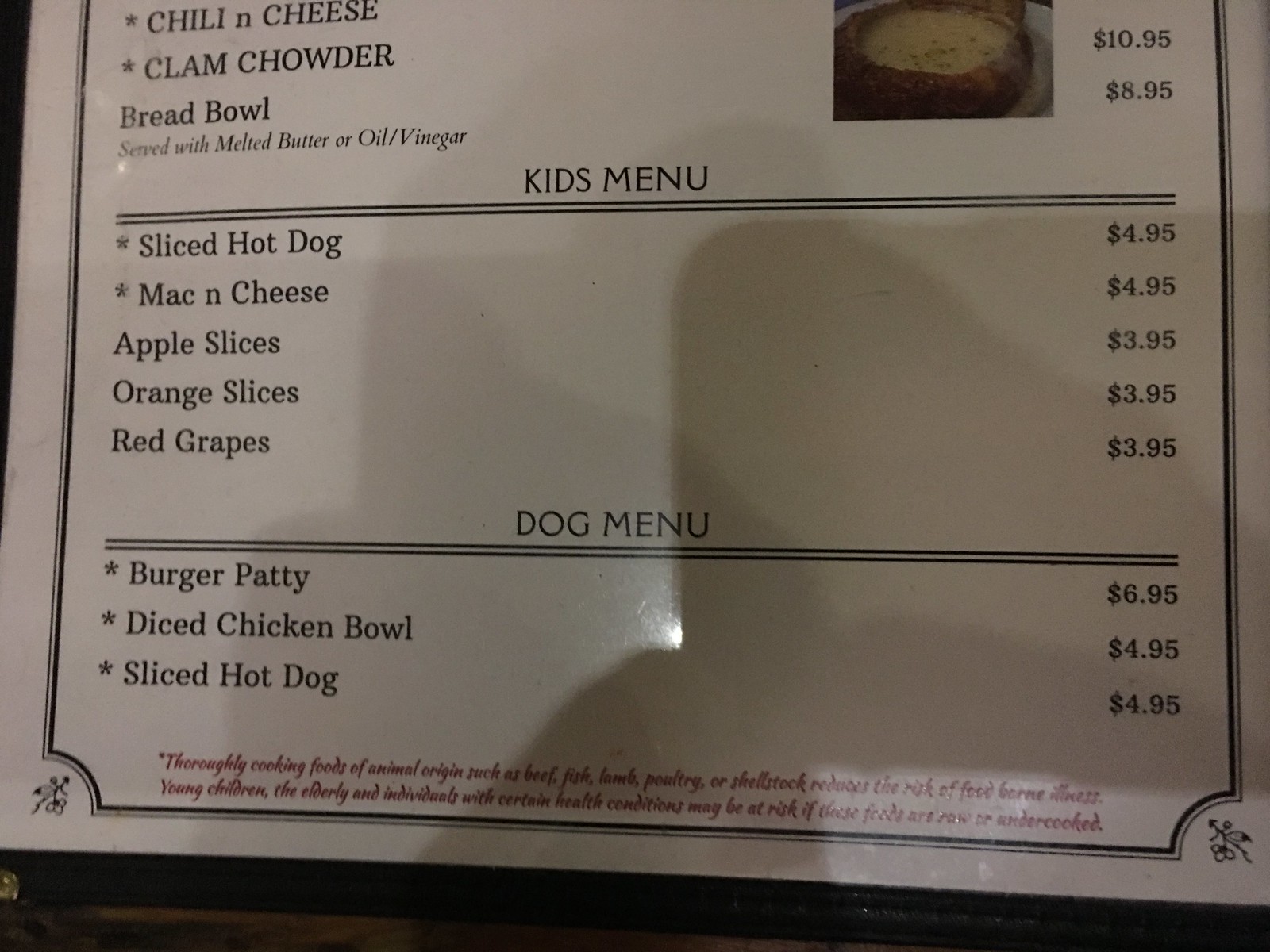This image showcases the lower portion of a menu set against a white background. Most of the text on this menu is printed in red. At the very bottom, an asterisked note reads: “Thoroughly cooked foods of animal origin, such as beef, fish, lamb, poultry, and shell stock reduce the risk of foodborne illness. Young children, the elderly, and individuals with certain health conditions may be at risk if these foods are raw or undercooked.”

Towards the top section visible in this image, the menu categorizes items under two distinct titles: "Kids Menu" and "Dog Menu." The "Kids Menu" offers a variety of child-friendly options including a sliced hot dog, mac and cheese, apple slices, orange slices, and red grapes. Adjacent to this, the "Dog Menu" features choices for canine companions, such as a burger patty, a diced chicken bowl, and a sliced hot dog.

Additionally, a minor part of another section can be seen at the topmost part of the image, showing an inviting picture of clam chowder served in a bread bowl.